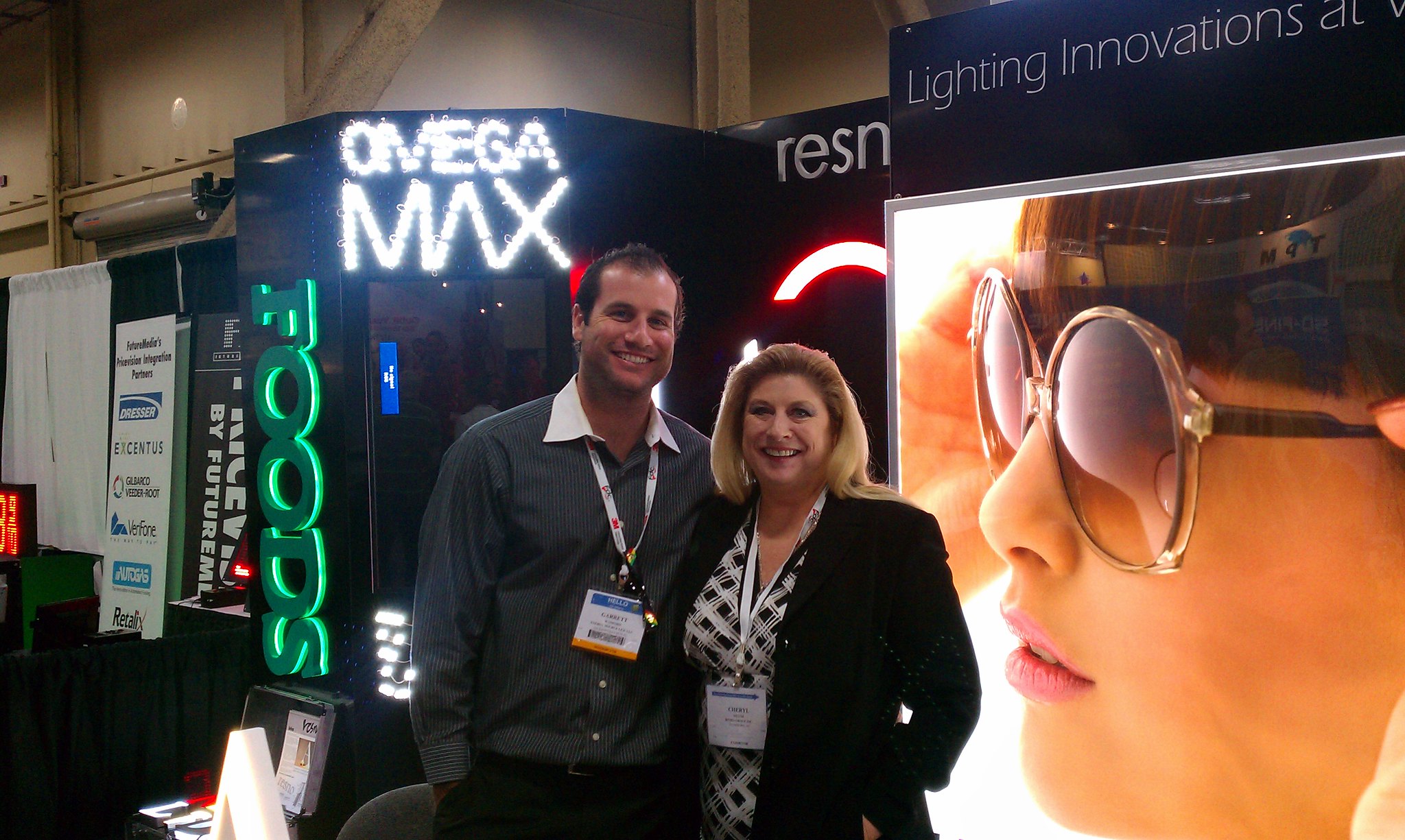In this vibrant image, a man and a woman stand closely together at what appears to be a convention or expo booth. The man, positioned on the left, has black hair slicked back and is wearing a gray long-sleeved button-down shirt with a white collar. A lanyard with a white card hangs around his neck, and his hand rests casually in his pocket. He smiles widely, while light reflects off his forehead. The woman next to him on the right has long blonde hair pulled back and is also smiling brightly. She wears a black coat over a black and white striped shirt, and she too has a lanyard with a card.

Together, they stand in front of a detailed booth backdrop. To their right is a glossy, high-contrast image featuring a woman's face in large brown sunglasses, with pink lips slightly parted. This image is topped with the words "Lighting Innovations" in a blue section. Moving left from this central image, the booth features more text and signage. The words "Omega Max" are prominently displayed in bright white lights, and beneath this, running vertically in green letters, is the word "Foods." Additional banners and flyers are visible, though their specifics are less clear. The overall scene suggests the booth is focused on lighting solutions, possibly related to food technology, and is decorated with various illuminated signs and promotional materials.